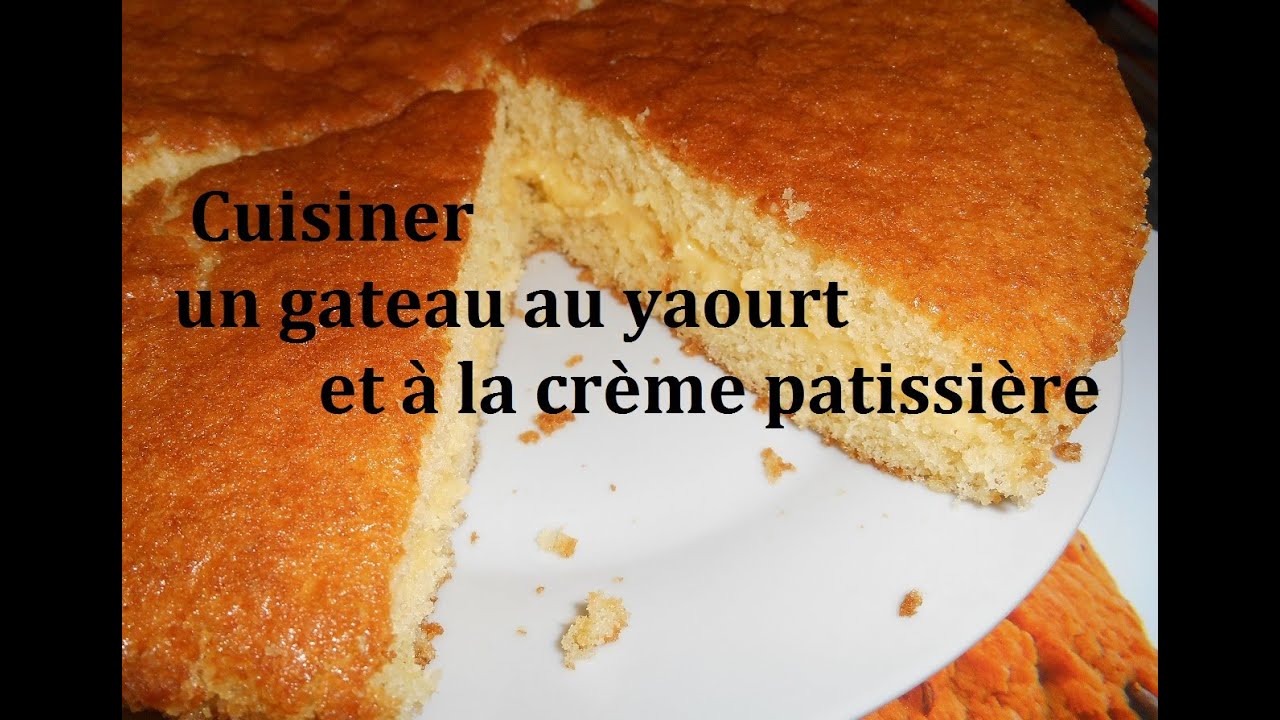The image is a color photograph featuring a layered cake on a white plate, with a thick brown edge framing the left and right sides of the photo. The cake has a beige top crust, and the body of the cake itself is white, with a layer of what appears to be yellow or white cream or custard in the center. The missing piece of the cake reveals some crumbs left behind on the plate, and another adjacent piece has been cut but not removed. There is also a suggestion of a large chocolate chip cookie beneath the cake. Prominently displayed over the image, in bold black lettering, is a caption in French that reads: “Cuisiner un gâteau à yaourt et à la crème pâtisserie,” roughly translating to “Cooking a yogurt and pastry cream cake.” The close-up perspective makes it difficult to determine the exact size of the cake.